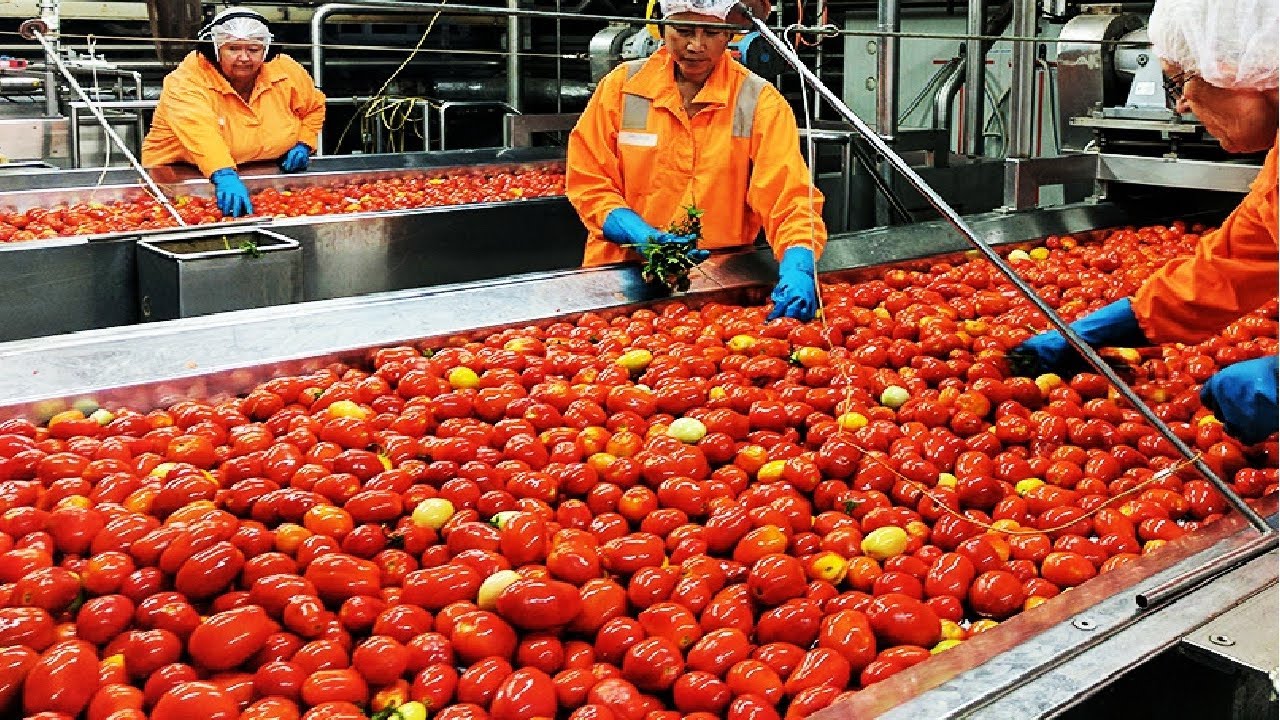The image captures a bustling scene at a produce processing plant, specifically dealing with Roma tomatoes. Three women, clad in orange jumpsuits with reflective strips, blue gloves, and white hairnets, work diligently at a large silver bin filled with overlapping red and a few yellow Roma tomatoes. They each wear earphones for communication or protection from noise. The workers are meticulously picking out leaves and other debris from the tomatoes, their hands buried in the vibrant pile. One woman in the foreground holds a bunch of green leaves she has removed, ready to dispose of them into a bucket nearby. In the background, complex silver machinery with conveyor belts and pipes weaves around, underscoring the industrial nature of the setting. The scene emphasizes the careful and thorough processing of the produce to ensure quality, with workers on either side of the line dedicated to their task.